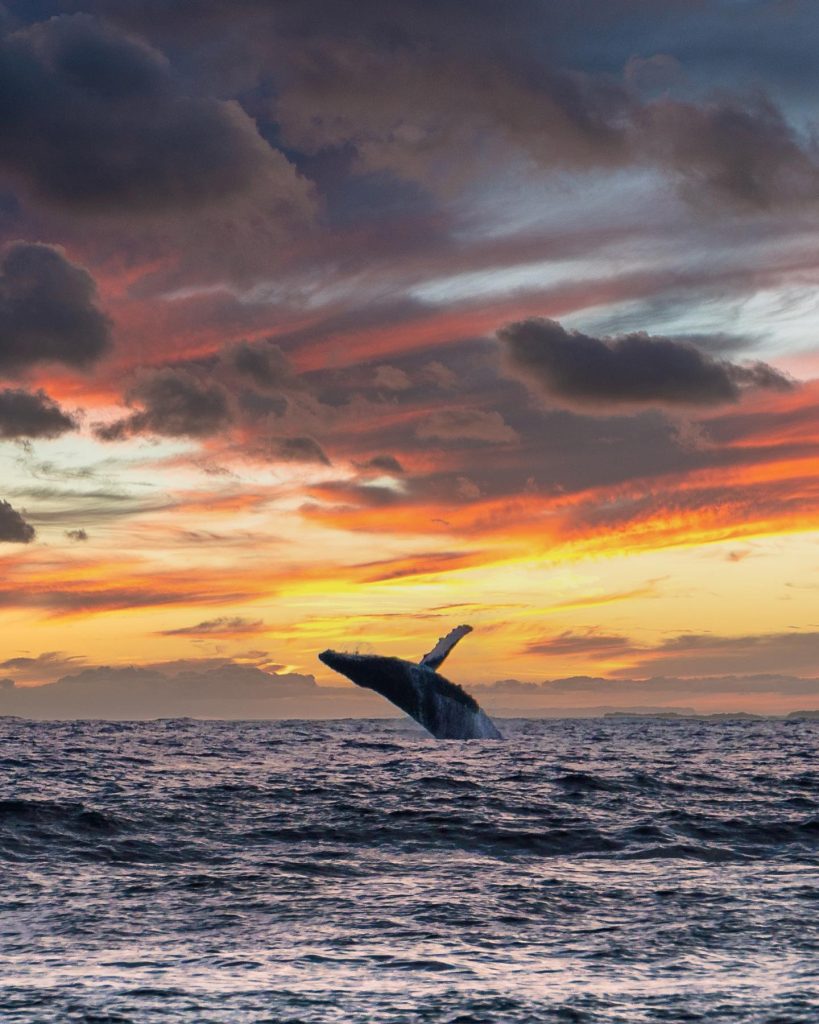In this evocative portrait-style image, a solitary humpback whale dramatically breaches the calm, expansive sea, its dark body arcing gracefully as its large fin extends skyward. The serene ocean, undisturbed except for gentle ripples and waves, stretches endlessly into the horizon. The sky above is a vivid tapestry of colors, starting with warm hues of orange and red near the horizon, indicative of either sunrise or sunset. These colors gradually blend into a yellowish tint, transitioning into a blue background interspersed with clusters of dark gray and gloomy clouds. Off in the distance, on the left-hand side, a faint outline of a mountain or island adds a subtle contrast to the vast seascape. The overall scene captures the awe-inspiring beauty and tranquility of nature, reminiscent of the majestic imagery from the classic movie "Free Willy."